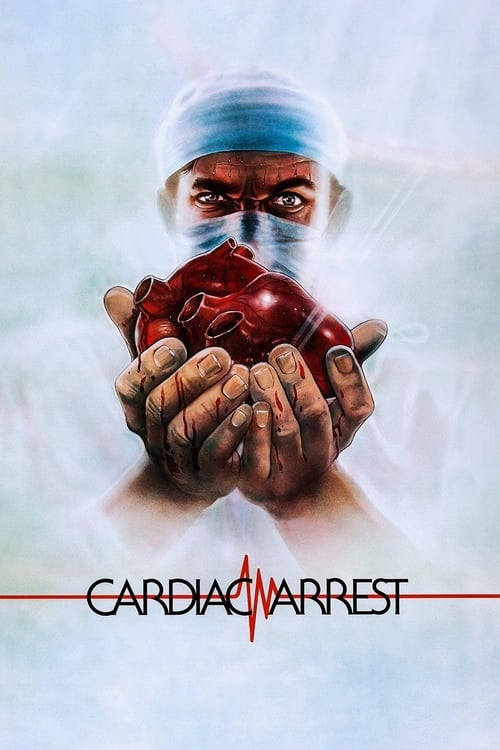The image is an artistic poster depicting a surgeon. The central figure, a man in blue surgical scrubs, including a hat and face mask, is holding a detailed, anatomically accurate human heart with blood streaking through his ungloved fingers. His serious expression is framed by deep creases on his forehead and piercing eyes that meet the viewer's gaze. The background has a blue, foggy quality that blends into the surgeon's figure, putting the focus squarely on him and the heart he holds. At the bottom of the poster, the text "Cardiac Arrest" is prominently displayed, intersected by a red electrocardiogram line that flatlines on both ends but shows a brief spike of activity in the middle.